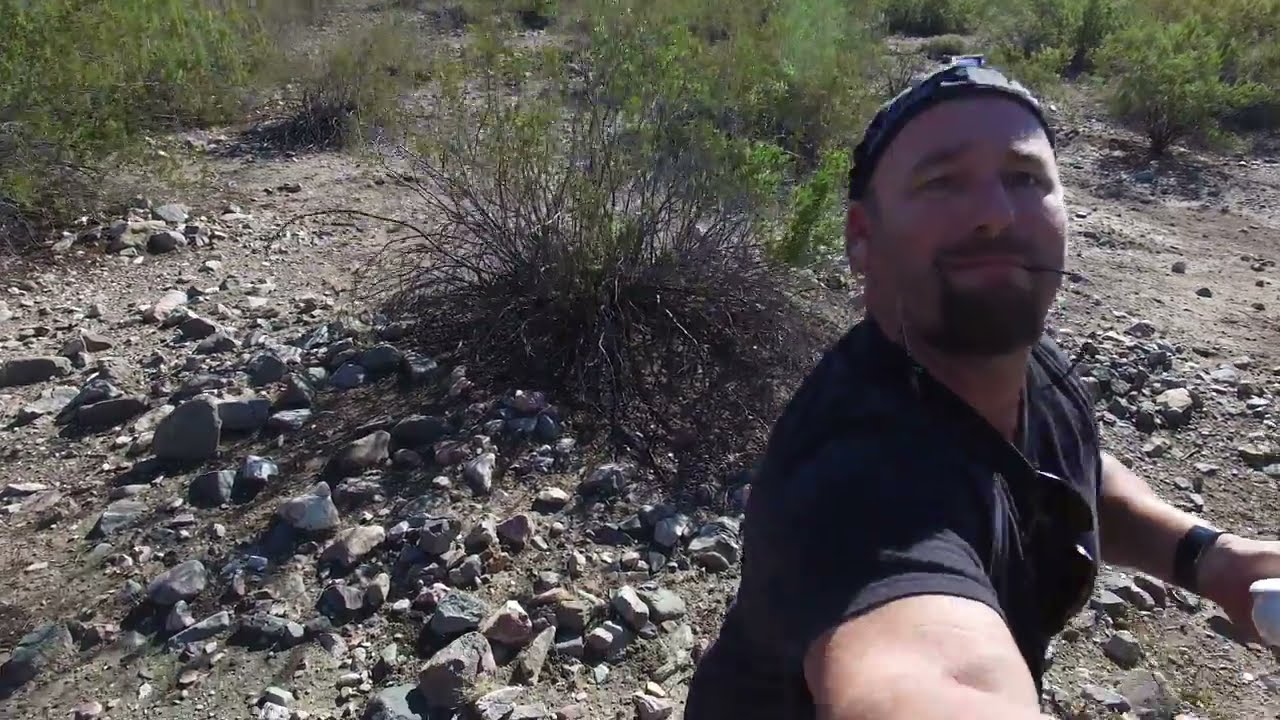The image depicts a bright sunny day in an arid, semi-desert landscape. From an aerial perspective, the viewer looks down on a rocky, dirt road that intersects with a paved road in the upper right-hand corner of the image. The dirt road, characterized by grooves carved out by water, extends downward to the left. Centered in the image is a white four-seat utility vehicle or golf cart, featuring a black and red trim and black wheels, and equipped with a white roof.

To the right of the vehicle stands a Caucasian man with a backward ball cap, dressed in a black short-sleeved shirt, black shorts, and dark sandals. He is holding a remote control for a drone and gazing upward towards the camera, which presumably is the drone he is controlling. Surrounding him and the vehicle are sparse, green, bushy shrubs.

In the lower right-hand corner of the image, a "Private Property, No Trespassing" sign lies on its side. The paved road in the upper right and the wild, sandy terrain populated with occasional bushes set a stark contrast, reinforcing the image's rugged, remote setting.